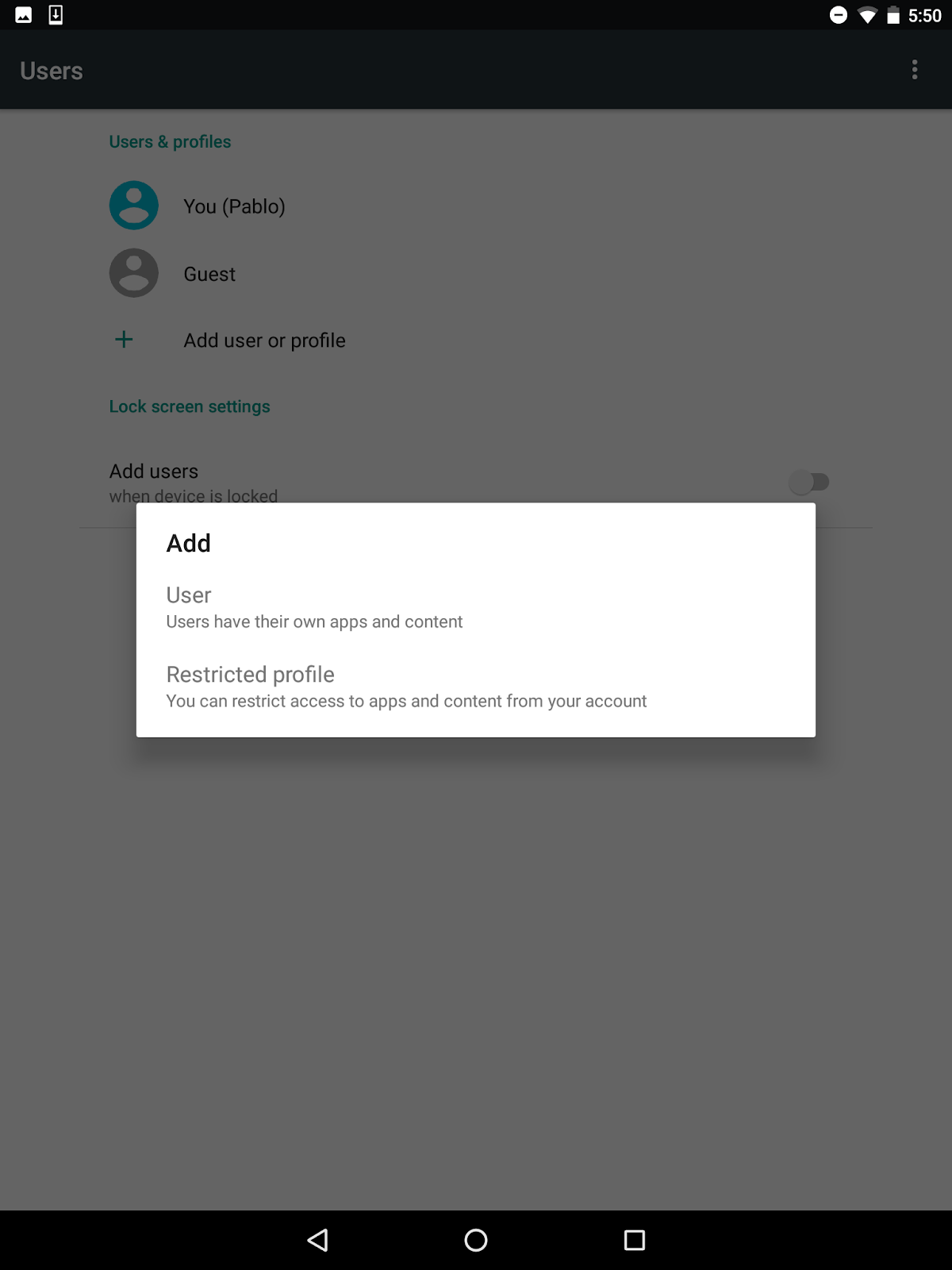This image is a screenshot of a phone displaying the "Users and Profiles" menu with a selection interface overlay. The background of the screen is grayed out, and a prominent white box in the foreground features the following text in black: “Add” in the upper left corner, followed by “User” below it. Underneath, the text explains, "Users have their own apps and content." Further down, it lists a "Restricted Profile," with the description, “You can restrict access to apps and content from your account.”

In the background, the topmost black bar displays status icons. On the left, there is a white box with black triangles followed by a download icon. On the right side, a white circle, nearly full Wi-Fi signal icon, and a battery icon with partial depletion are visible, along with the time displayed as 5:50.

Below this, another black bar contains the text "Users" in white capital letters on the left, and three horizontal dots on the right for additional options. The section below this bar is white and prominently shows "Users and Profiles" in green text. Here, represented icons include a blue circle with a white silhouette labeled “You (Pablo)” and a gray circle with a white silhouette labeled “Guest.” Further down, a green plus symbol paired with the text “Add User or Profile” indicates an option to add new users.

Additional options listed below this include "Lock Screen Settings" and "Add Users when device is locked." At the very bottom of the screen, a final black bar showcases three central icons: a play triangle on the left, a circle in the center, and a square on the right, resembling typical navigation buttons.